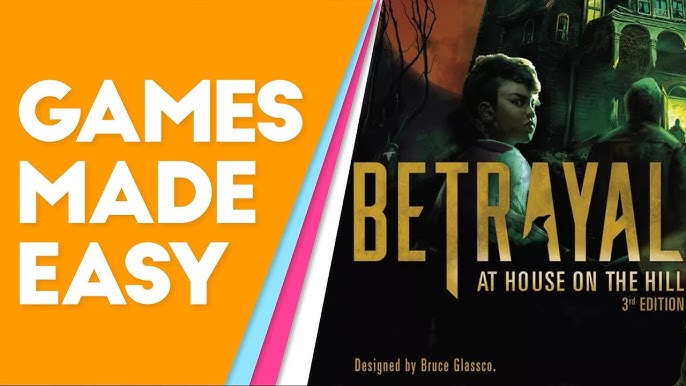The image is an advertisement banner that is split diagonally, featuring both text and an illustration. On the left half, against an orange background, white text boldly states "Games Made Easy." Separating this section from the other are three diagonal lines in blue, pink, and white. The right half of the banner showcases a creepy night-time scene with an old, dark Victorian house that evokes a horror atmosphere. The sky is ominously orange, while the rest of the scene is cloaked in night’s darkness. Two characters are depicted: a little boy looking back anxiously, and an older man, portrayed in black shadow, walking towards the house’s green-lit door. Prominently featured in gold, stylized text is the title "Betrayal at House on the Hill, 3rd Edition," with the black crow cleverly positioned in the "A" of "Betrayal." Smaller text below credits Bruce Glasgow as the designer.